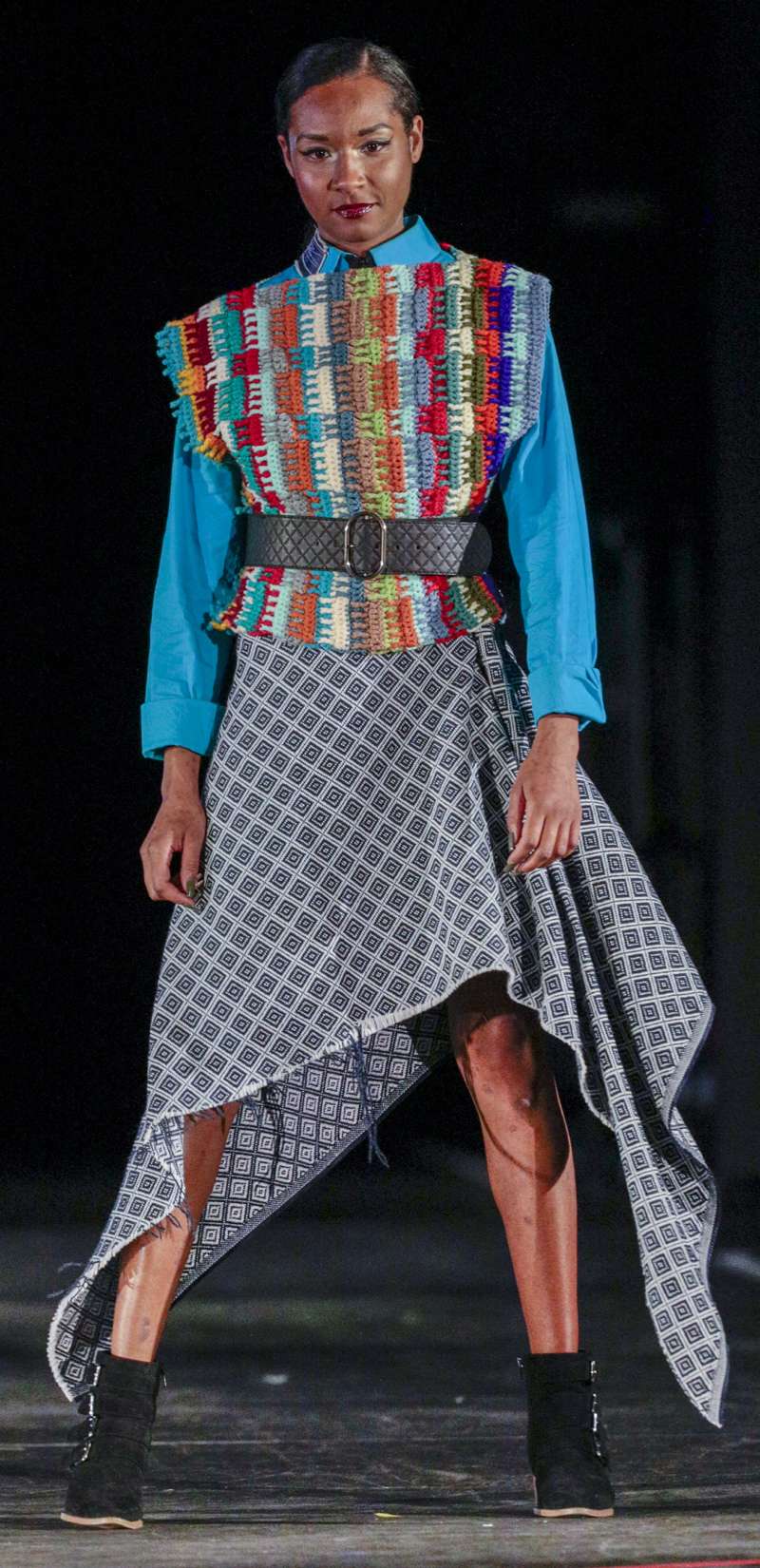A striking model is confidently posing on a dark gray runway, showcasing a bold and eclectic ensemble. She has sleek, parted short black hair and captivating brown eyes. Her attire begins with a collared, long-sleeved blue blouse, the sleeves slightly rolled up, providing a structured base. Over this, she wears a unique vest featuring an eye-catching quilt-like pattern in vibrant hues of blue, orange, red, and white. The vest is cinched at the waist with a stylish black belt, emphasizing her silhouette. Her skirt is a long, light gray piece adorned with a repetitive pattern of gray and black squares, intricately designed to swoop up towards one thigh, revealing her knees while cascading down elegantly at the sides. Completing her look are short black ankle boots, adding a touch of edge to her polished appearance. The model's poised stance, with legs slightly apart and hands at her side, exudes confidence and grace, perfect for the runway setting.